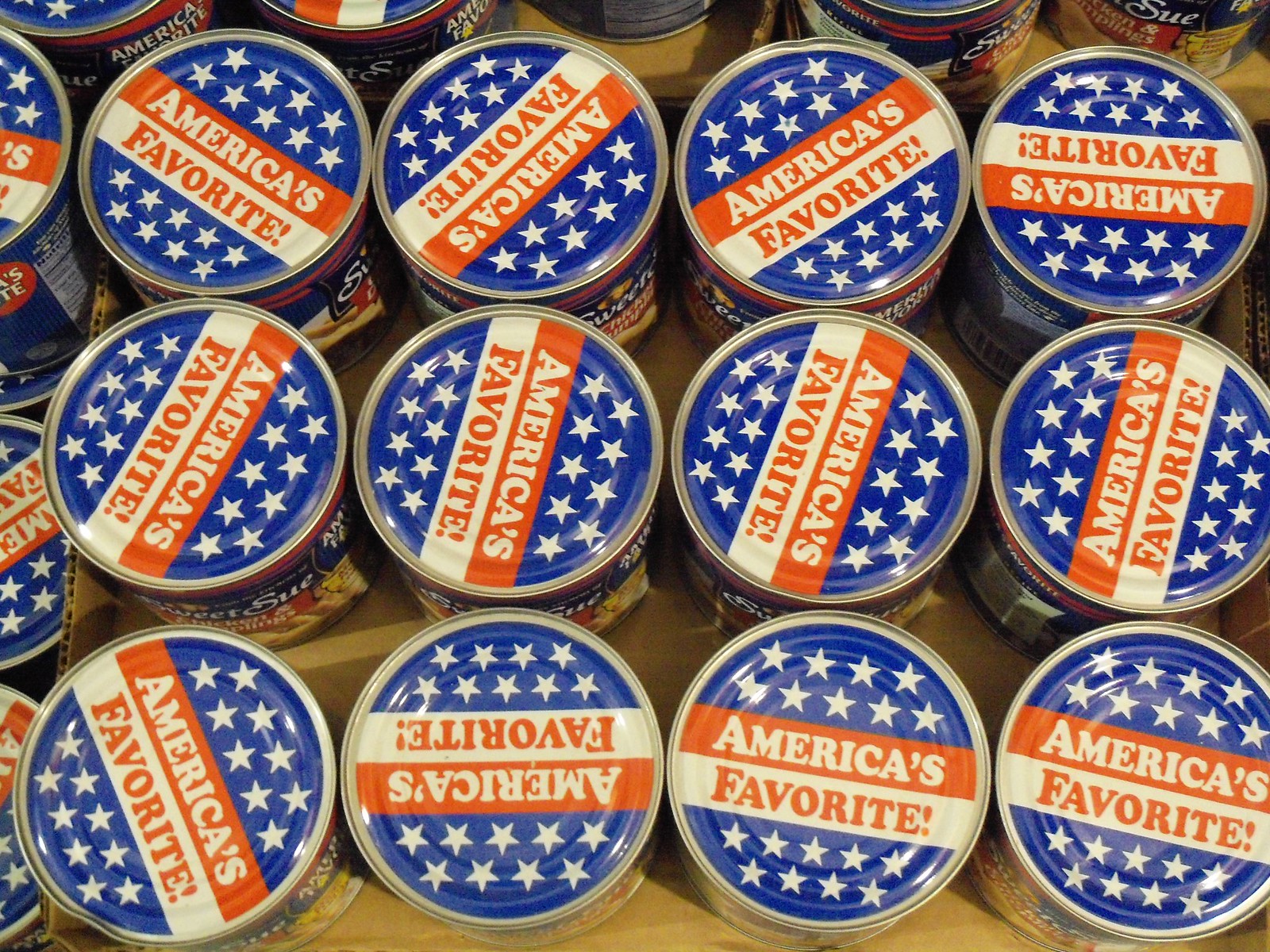This color photograph, taken from an overhead perspective, features a neatly arranged collection of 20 metal soup cans, placed in a brown cardboard container. Each can is designed with a patriotic theme: the top and bottom sections have a blue background adorned with white stars—18 stars in total, with rows of 4, 5, 5, and 4. A red stripe runs through the middle of the can, displaying “America’s” in white lettering, while a white stripe beneath it has “Favorite!” in red lettering. While portions of some cans are cropped from view, each visible can is identical to the next. Despite the inability to see the full labels due to the overhead angle, there's an indication that one label might read "chicken and dumplings."